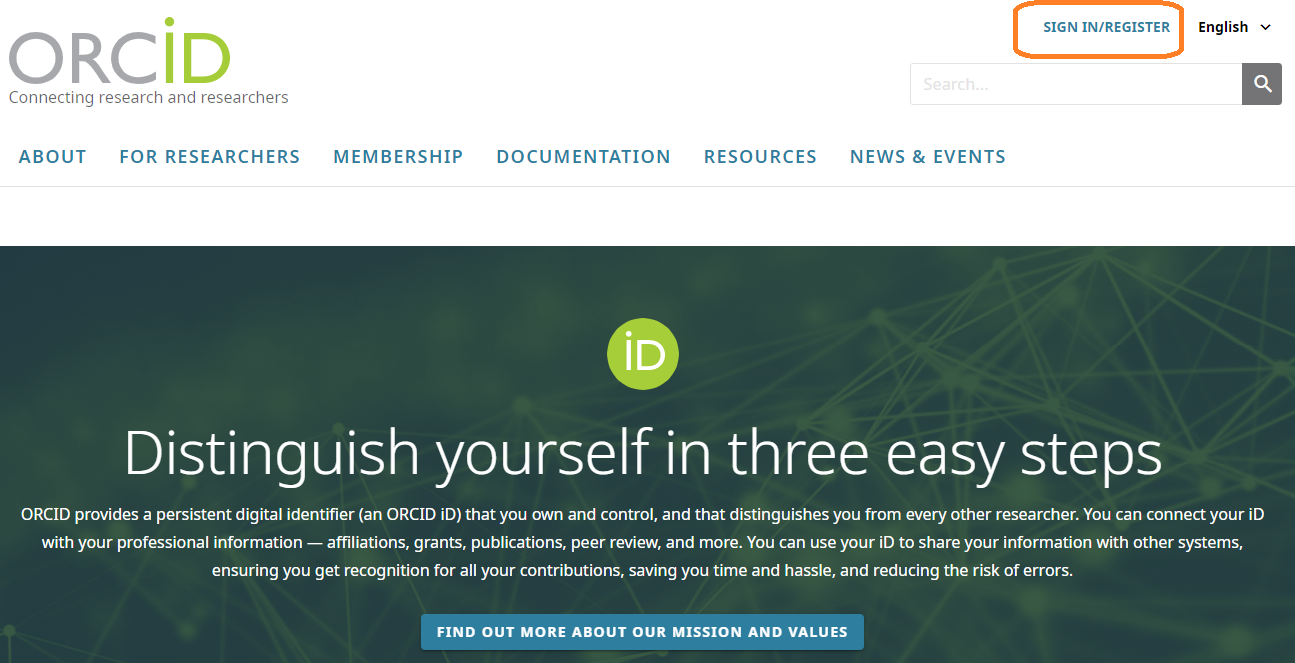The screenshot features a section of the ORCID website. At the top, there's a white background with the ORCID logo prominently displayed on the left. The logo consists of the letters "ORCID" where "O-R-C" is in gray and "I-D" is in a lime green color, with the "I" being lowercase yet proportionately tall with a dot on top.

On the right side of the header, "Sign-In/Register" is written with an orange border around it, and next to this, "English" is displayed in bold, dark print with a capital "E" and an accompanying dropdown menu. Below this section, there is a search bar characterized by a charcoal gray square containing a white magnifying glass icon.

Further down, a navigation bar features blue, capitalized text for links such as "About," "For Researchers," "Membership," "Documentation," "Resources," and "News and Events," spanning from left to right.

Beneath the navigation bar, a banner displays a network-like graphic with connecting dots and fiber-optic lines. At the center of this graphic is a lime green circle with the letters "I-D" in it. Surrounding the circle, in white text, it reads: "Distinguish Yourself in Three Easy Steps." Finally, at the bottom of the screenshot, another blue banner with white text invites users to "Find Out More About Our Mission and Values."